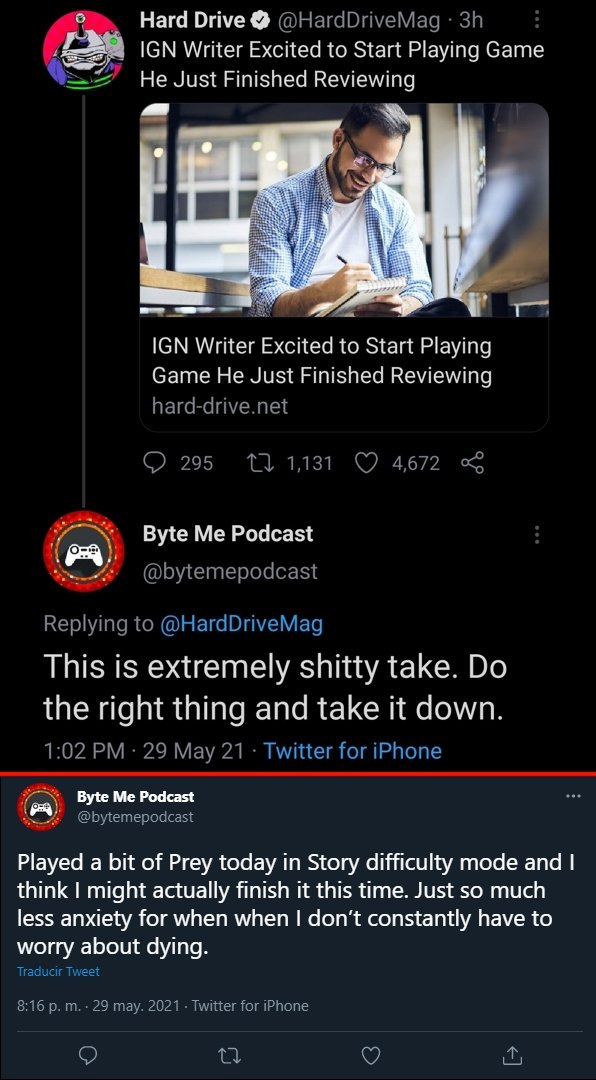Here is a detailed and cleaned-up caption for the image:

---

The image is a screenshot of a Twitter post dated May 29, 2021, at 1:02 PM, taken from an iPhone. The post features two main elements side-by-side. On the left, there is an article from "hard drive net" showing a man with glasses, wearing a button-down long-sleeved shirt, writing in a notebook. The headline of the article reads: "IGN writer excited to start playing game he just finished reviewing." To the right, there is a profile picture contained within a red circle, depicting a character that looks robotic. The Twitter post this article was shared from is associated with the "Bite Me" podcast, which has provided a critical commentary on the article. Their tweet above the shared article states: "This is an extremely shitty take, do the right thing and take it down."